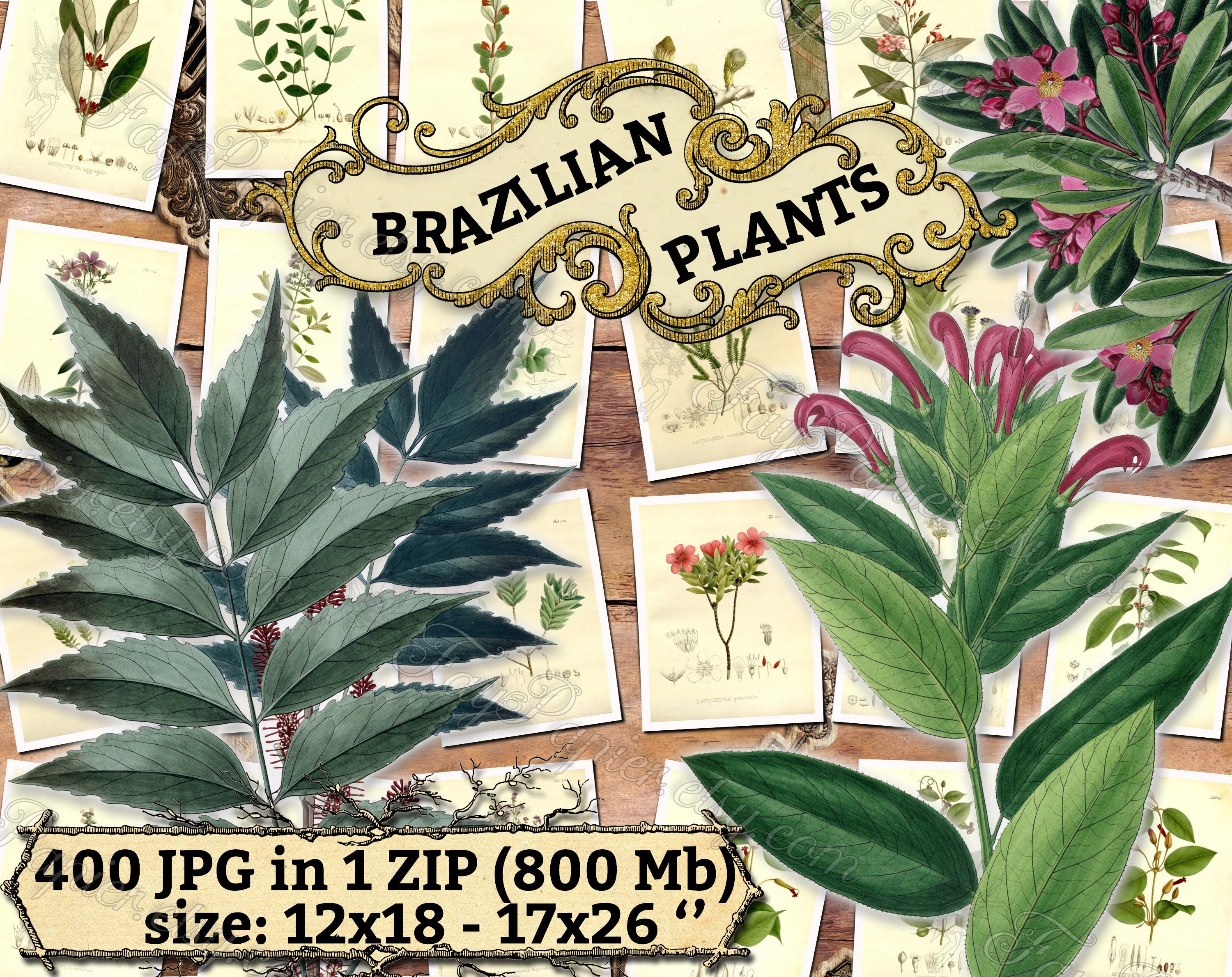The image is an advertisement for a digital graphic design collection titled "Brazilian Plants." The center of the image features the title in bold, black capital letters within a whimsical, gold-bordered, beige cloud-like shape. Surrounding this central element are detailed illustrations of various Brazilian plants. These drawings are depicted on postcard-like cards, creating a layered effect that includes overlapping larger plants with vibrant green leaves, purple flowers with yellow centers, and some pink flowers. The background resembles a brown wooden plank, enhancing the natural theme. At the bottom left of the image, text indicates that the collection is available as a "400 JPEG" file within one zip archive, totaling 800 megabytes, with dimensions ranging from 12 x 18 inches to 17 x 26 inches. A watermark overlays the entire picture, signifying that this is a stock photo.